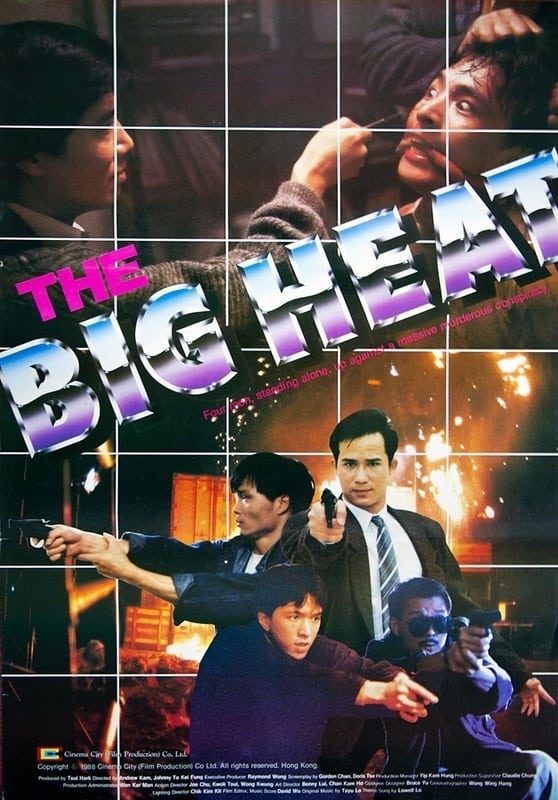The movie poster for the Asian film "The Big Heat" features a striking blend of color photography, graphic design, and typography. At the top of the poster, "The Big Heat" is written in bold white English text. Vertically aligned Asian characters, rendered in black, appear between the words "Big" and "Heat." The background is dominated by a blue sky with billowing white clouds and a curving bridge that recedes into the distance.

In the upper left, two men in black suits are dramatically leaping atop a train, their image posterized in high-contrast black and white. Below the Asian characters, four men stand side by side at the bottom center of the poster. The man in the center is rendered in full color, wearing a dark gray business suit, a white shirt, and a blue striped tie. He holds an object by his side and has one hand in his pocket. The other three men are portrayed in stark black and white, giving them a menacing, mobster-like appearance. The man on the far left sports sunglasses, a small mustache, a black jacket, and white pants. The two men to the right of the central figure wear black jackets, with the one on the far right featuring white stripes and cuffs. This visually compelling poster utilizes a combination of photographic techniques, special filters, and illustration to create a captivating and dynamic composition.